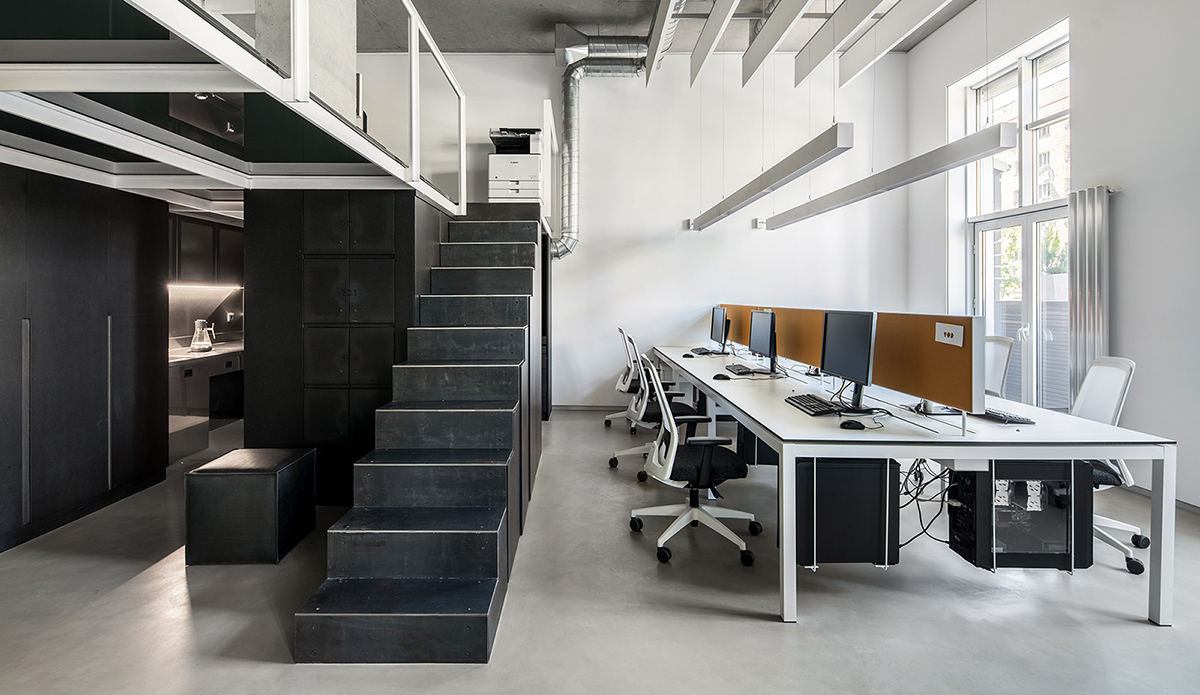The image depicts a modern office space characterized by a large, white, rectangular table situated in the center with six computer workstations—three on each side. Each workstation consists of a computer monitor, keyboard, and mouse, with accompanying black office chairs. The table also supports cork boards between the computer setups. Above the table, there are long, white rectangular lights hanging from the ceiling, illuminating the room which also benefits from natural sunlight streaming through side windows. 

On the right side of the room, there is a glass door with a white frame, adding to the office's modern aesthetic. The wall housing the door is complemented by additional glass windows above it. In the left center of the image, a set of large, black steps without railings leads to a loft area that appears to house a copy machine. The structure of the steps and the lack of visible floor upstairs contribute to a sense of minimalistic design. Below the loft, to the left of the stairs, a small pocket room with black walls and lighting suggests a potentially cozy or private space. 

In the downstairs area, next to the large table, is a kitchen area marked by a coffee urn among other typical kitchen fixtures, seamlessly blending functionality with the office's sleek design. The entire composition, featuring white walls, modern fixtures, and sleek furniture, gives the room a clean, high-tech feel, possibly hinting at creation via an augmented reality program.